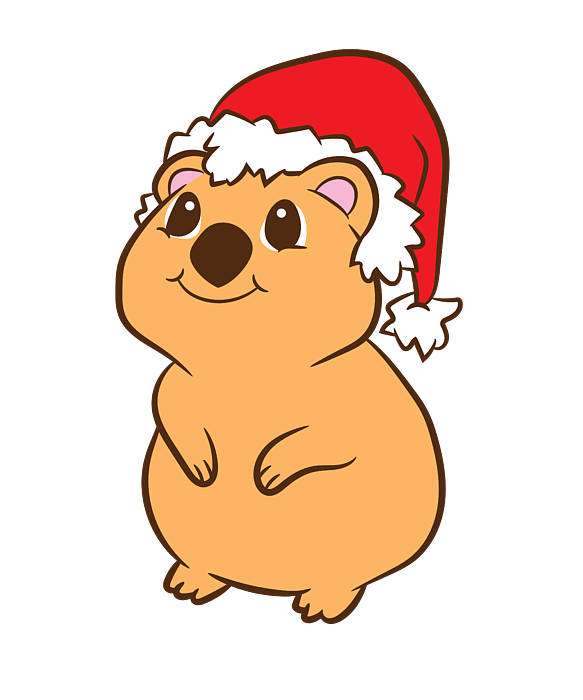The image depicts an adorable cartoon drawing of a koala, characterized by a thick, dark brown outline. The koala features a round head with large, expressive brown eyes and a prominent, bulbous, brown nose. Its ears are round with pink interiors, adding to its charming appearance. The character displays a cheerful smile that stretches from cheek to cheek. The koala’s body is similarly round and beige or camel-colored, matching the head in size, and has short, stubby limbs with visible toes outlined in brown. This endearing koala is adorned with a festive red Santa hat, complete with white fur trim and a dangling, fluffy white ball at the hat's tip, enhancing its joyful and celebratory look.